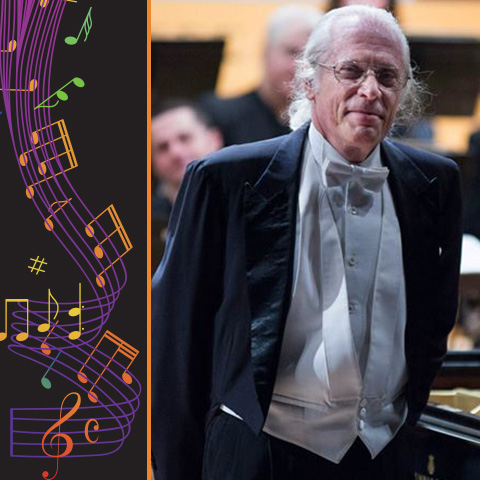The composite image consists of two distinct sections: a colorful illustration on the left and a close-up photograph on the right. The left section occupies about one-third of the image and features a vibrant depiction of music with lines like those on sheet music. Various musical notes, colored blue, yellow, orange, and green, appear to be floating through the air against a purple staff, creating a sense of movement.

The right section is a photograph of an elderly white man, possibly a conductor or musician, shown from the waist up. He has white hair pulled back into a ponytail and is partially balding. He wears round wireframe glasses and is dressed formally in a navy blue tuxedo with a white vest and a white bow tie over a button-up shirt. He sports a pleased expression on his face, with a backdrop that hints at an orchestra setting with other musicians slightly visible behind him. The detailed illustration and the photograph together create a rich visual narrative of music and its conductor.